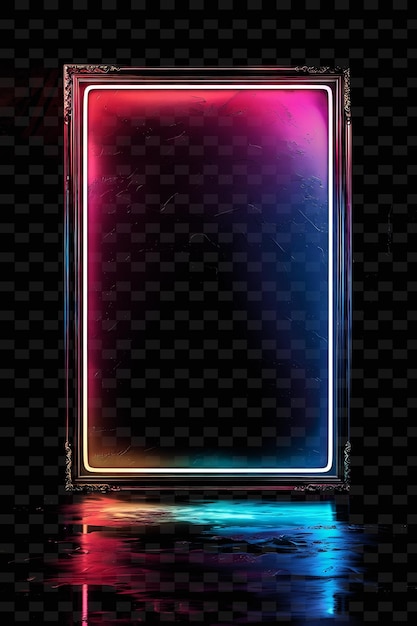This image captures a large, intricately carved rectangular picture frame made of dark wood, standing against a checkered wall composed of black and charcoal gray squares. The frame, positioned vertically, is empty, allowing the background to be visible through it. Adorned with LED neon lighting on its perimeter, the frame emits a striking display of colors: a vibrant magenta pink on the left and upper sides, and an electric cool blue on the right and bottom sides. The neon lights cast their hues onto the interior of the frame, creating a dynamic visual effect. Shadows and reflective patterns from the LED lights grace the floor below, mimicking the colored lights as if mirrored in water, enhancing the contemporary and artistic ambiance of the scene.